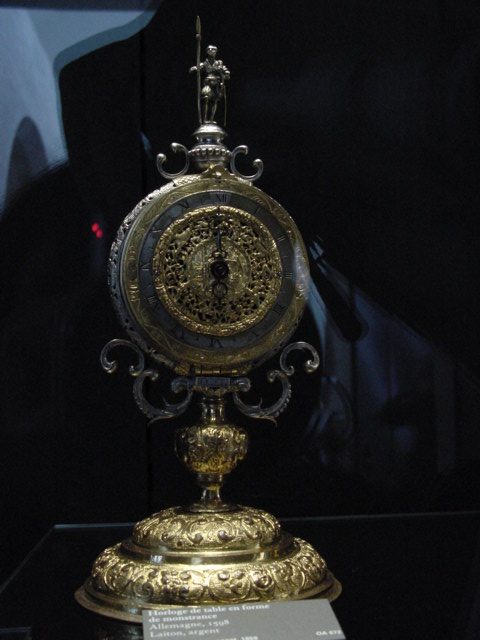In the image, a trophy standing prominently on a sleek black platform captures the viewer's attention. Beneath the trophy is a gray business card adorned with white horizontal lettering. The trophy's base is a striking gold, comprising two gold circular platforms. Advancing upwards, the design features intricate, curvy, gray-like vines. Above these vines, there's a circular pattern exhibiting alternating colors of gray and gold, culminating in a gold circle at the center. Crowning this intricate design are two open silver rings, leading to the statue of a small person positioned at the very top. The background melds shades of black and light blue, creating a striking contrast that accentuates the trophy’s elegance.